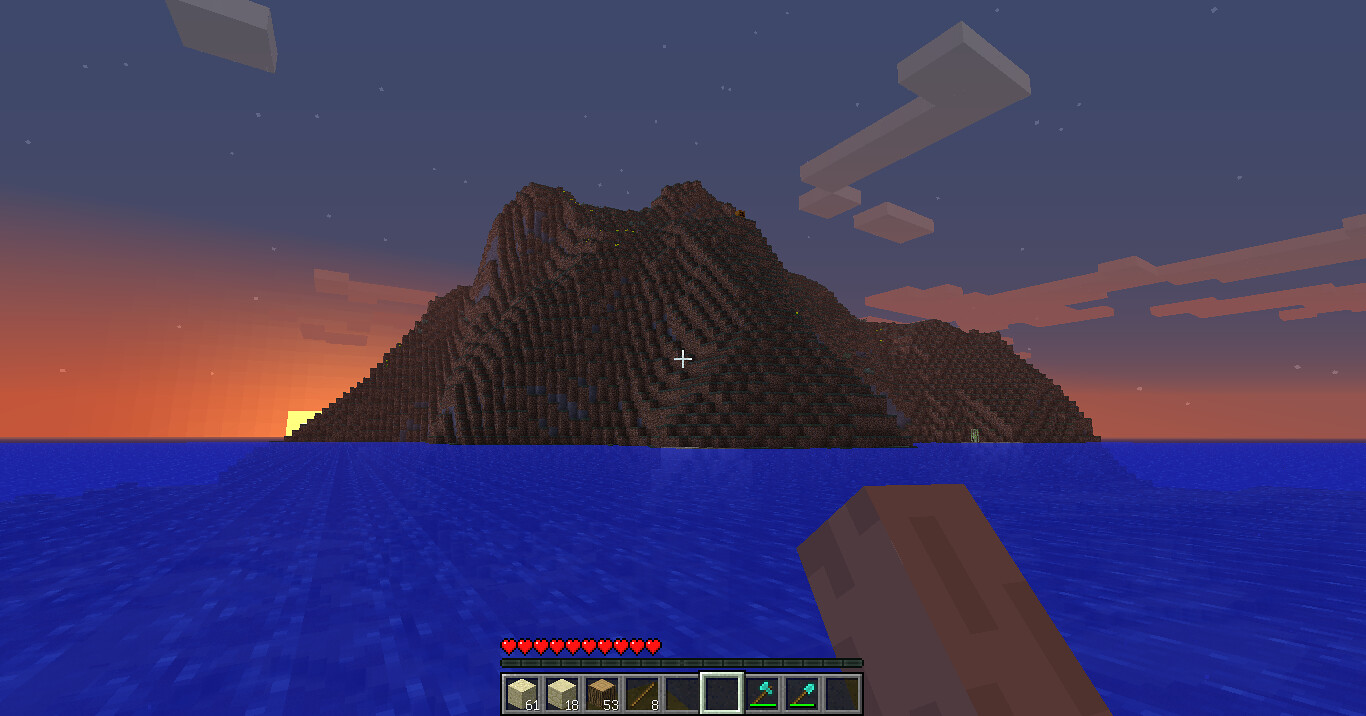This is a detailed screenshot from the video game Minecraft, featuring a geometrically-styled animation. The central focus is a large, dark gray island made up of thousands of small rectangular cubes, possibly representing a mountain or volcano. This island is set against a backdrop of a vibrant sunset, with the sky transitioning from bright pink to periwinkle blue. Block-like clouds float above, adding to the distinctive geometric aesthetic. The ocean beneath the island is bright blue, with lighter blue geometric patterns composed of long straight lines and small squares. In the foreground, there appears to be a faint outline of a gun or sword partially submerged in the water. At the bottom of the screenshot, there's a menu bar displaying a line of 10 hearts that represent the player's health, alongside various inventory items, including blocks with quantities and tools.